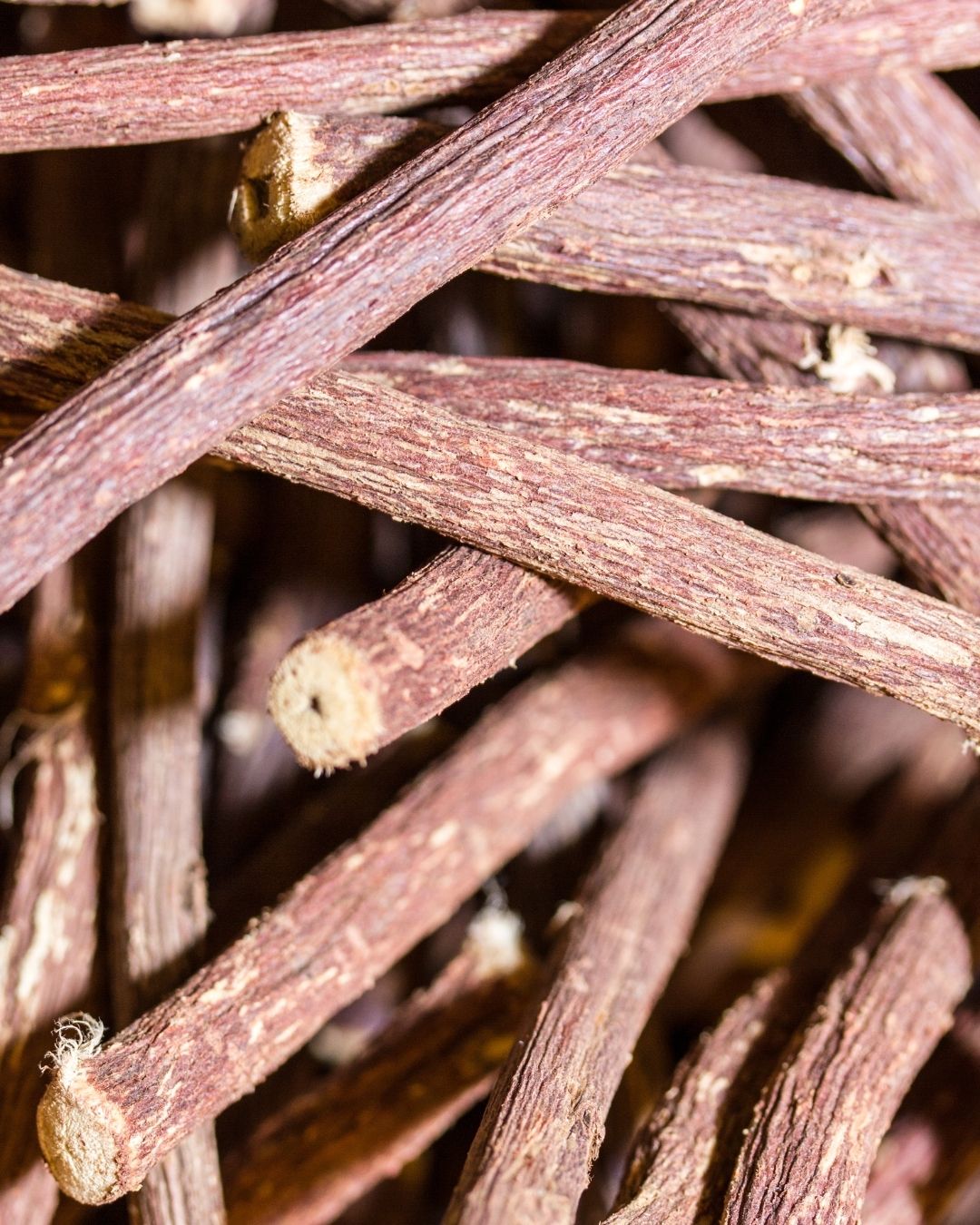This image is a close-up of numerous brown sticks with a wrinkled, grooved bark and nicked-off pieces, revealing white, pulpy interiors. They are crisscrossed and stacked at various angles, forming a dense, chaotic pattern. Some sticks have perfectly sliced-off ends, exhibiting light brown, circular sections with tiny holes or hollow areas in the center. The sunlight reflects off the sticks, highlighting the intricate textures and shadows. The top layers are more in focus, while the others blur into the background. No other objects are visible, and the entire view is dominated by the intricate layout of the sticks, which resemble a disorganized pile of natural, wooden debris.